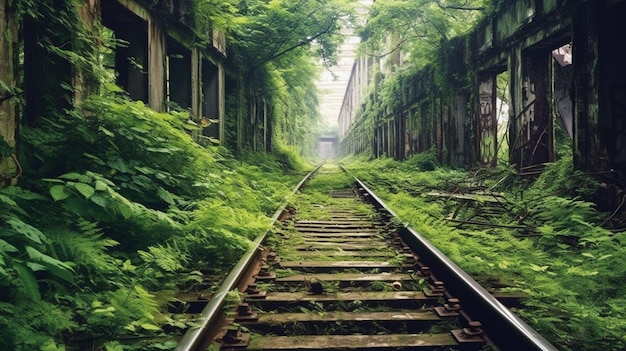In this colored photo, the camera is positioned in the middle of an overgrown, seemingly abandoned train track, capturing a straight path that narrows into the distance. The rails, showing signs of disuse with greenery sprouting through the slats and over the tracks, suggest that trains have not passed through in a long time. Flanking the tracks are dilapidated structures, possibly old factories or homes, recognizable as two or three-story buildings with broken windows and open doorways. These buildings are overrun with trees and vegetation, further evidence of neglect. The scene is framed by walls and railings, and way down the track, a small overhead bridge appears faintly in the distance, partially obscured by the dense foliage reclaiming the area.